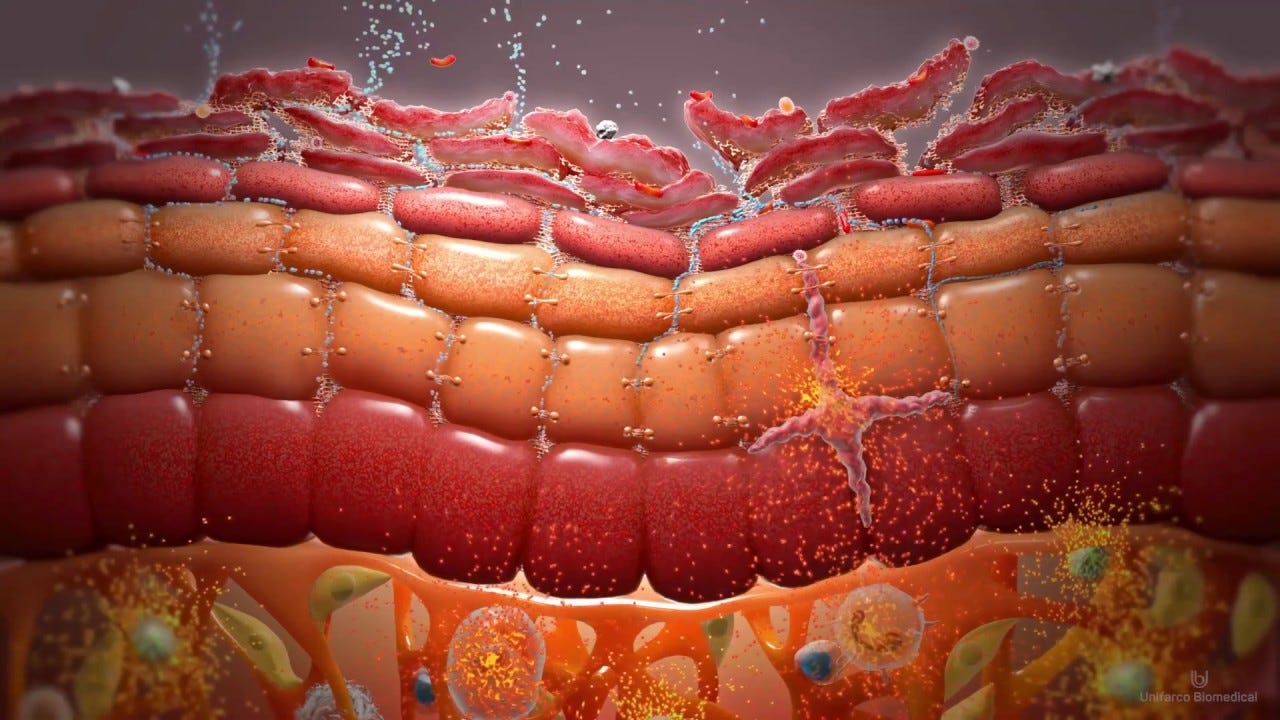The image appears to be an abstract, possibly computer-generated artwork or a highly stylized photograph. The scene is an intricate design featuring a medley of objects and shapes that resemble a vibrant mix of tiles or ceramics. At the bottom, there are numerous small, glazed, and colorful tiles, reminiscent of stones or gumdrops, in shades of red, cream, orange, blue, and green. These resemble the shape of teeth or chiclets gum. Above this section, there are elongated, cylindrical shapes that vary in color, resembling hot dogs or bacterial forms, which transition into a layer of shapes that look like slices of bacon. This whole composition appears to have a liquid element to it, as there seem to be bubbles and particles floating around, giving the impression of being underwater. The background is primarily a neutral gray, which helps the medium-toned, multicolored elements stand out without being overly vibrant.